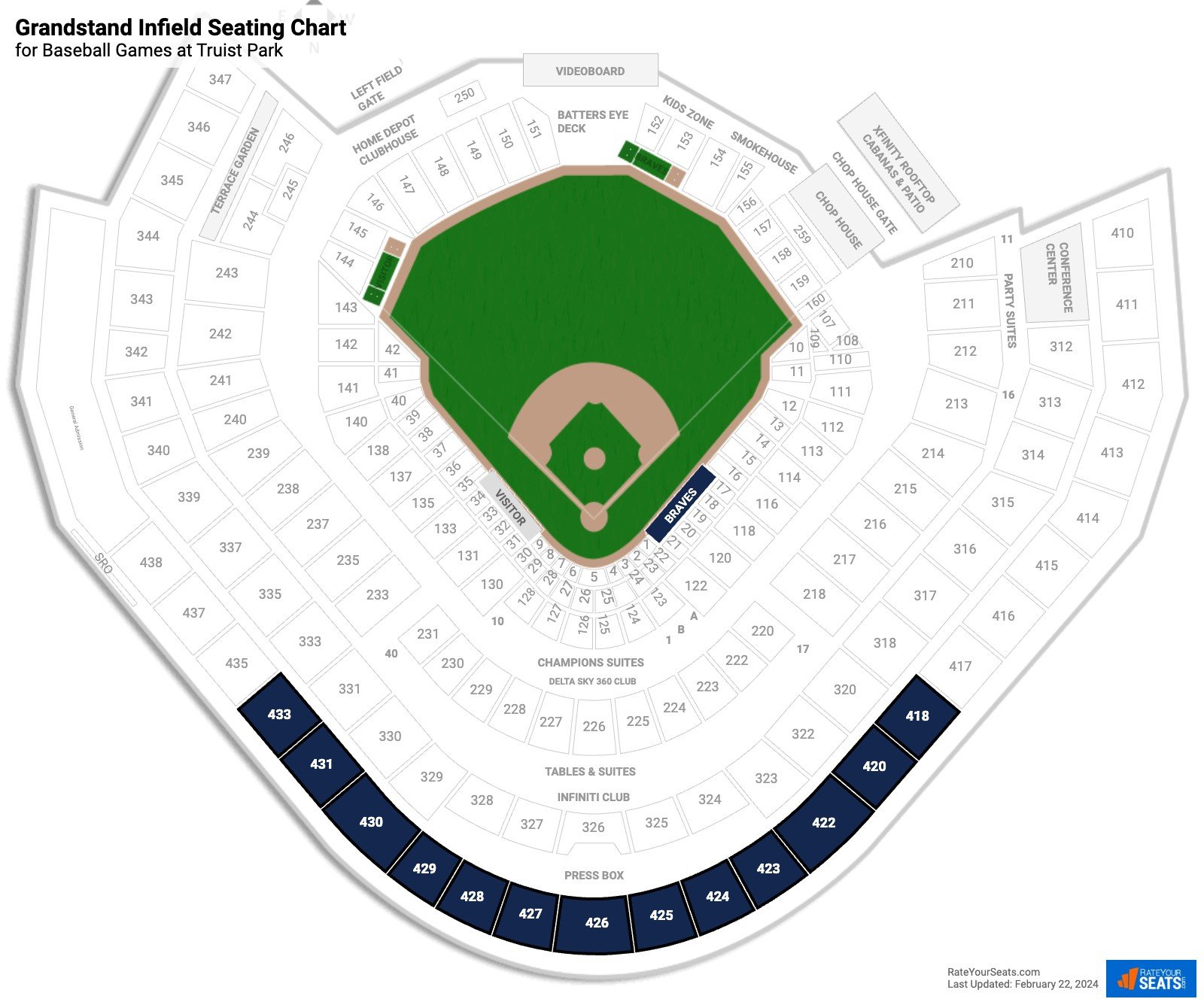This is an aerial seating chart for Truist Park, home of the Atlanta Braves, specifically highlighting the Grandstand Infield section. The stadium's seats are mostly depicted in white, with select sections in color, providing a contrast that draws attention to specific areas. The vibrant green baseball field dominates the center of the image, encircled by a lighter brown infield and warning track. 

Surrounding the seating area is a distinctive thick gray border, though no additional boundaries mark the outer edge of the field. In the top left corner, bold black text reads "Grandstand Infield Seating Chart, for baseball games at Truist Park." Beside the field, a blue diagonal box with white font spells "Braves" on the right, while a gray box with gray lettering reading "Visitor" appears to the left. Above the outfield, green boxes are highlighted, indicating special areas.

At the very top of the image, a semi-circular arrangement of blue boxes, likely representing premium suites or sections, is numbered from 418 to 433. These boxes are situated at the highest point of the stadium, above the press box. At the bottom, the image is subtly branded with a watermark in gray that states "RateYourSeats.com," and it includes the text "Last Updated February 22, 2024." Additionally, a blue icon with an orange logo and white lettering appears, adding a final touch of detail.